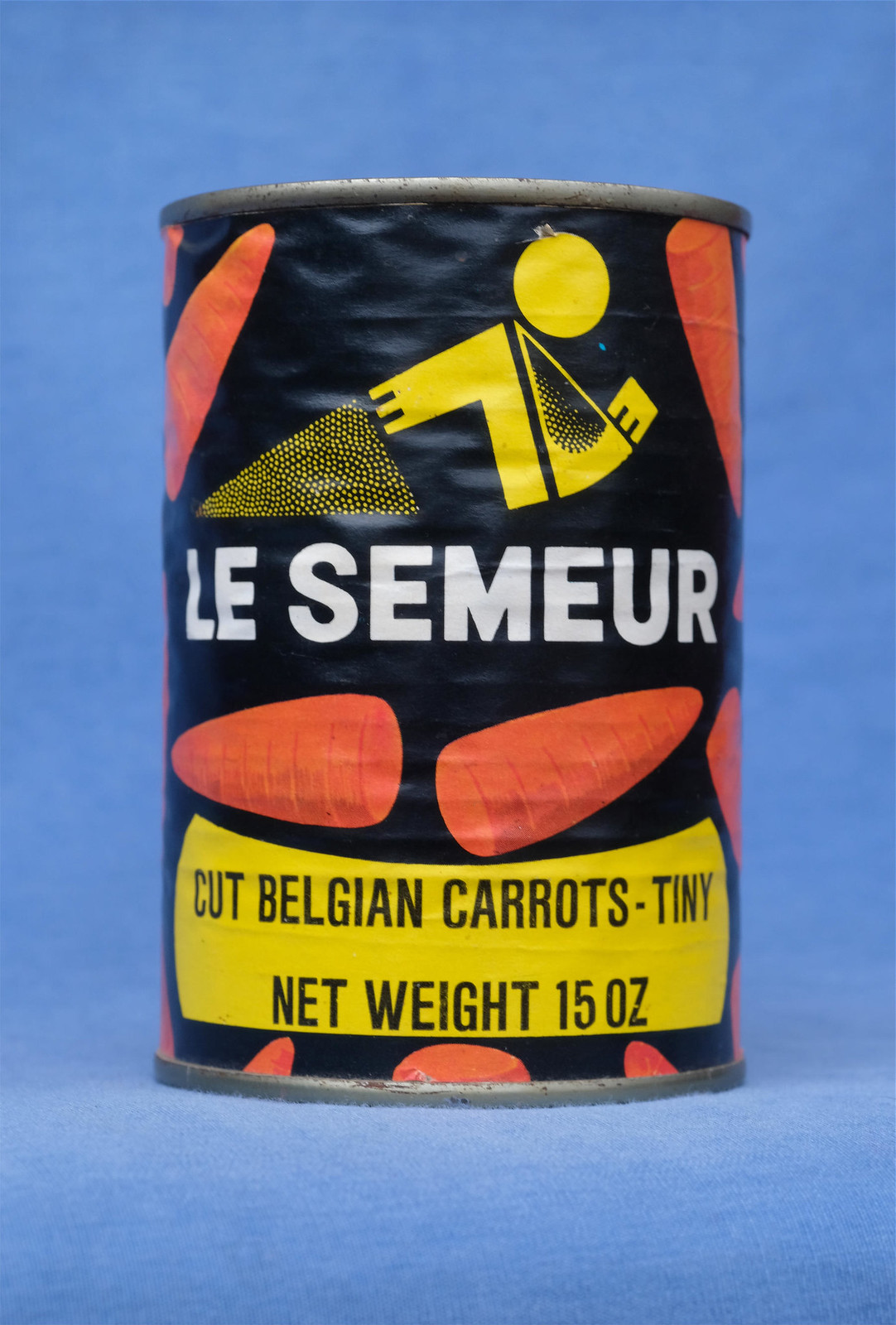This detailed vertical rectangular image against a medium blue background features a black-labeled can of carrots. The can prominently displays the words "LE SEMEUR" in large white capital letters in the center. Beneath this, an array of baby carrots, depicted with one pointing left and another slightly longer one pointing right, are illustrated vividly. The top section of the can label has a distinctive yellow, almost curved rectangular area with black all-capital letters stating "CUT BELGIAN CARROTS - TINY," followed by "NET WEIGHT 15 OZ." Additionally, on the right side of the can, there is a yellow figure resembling a block-man with vertical stripes indicating arms, a black shirt, and a small dotted triangle near the hand. The detailed artwork of the yellow figure and multiple small carrots, alongside critical textual information, completes the sophisticated design of the can’s label.